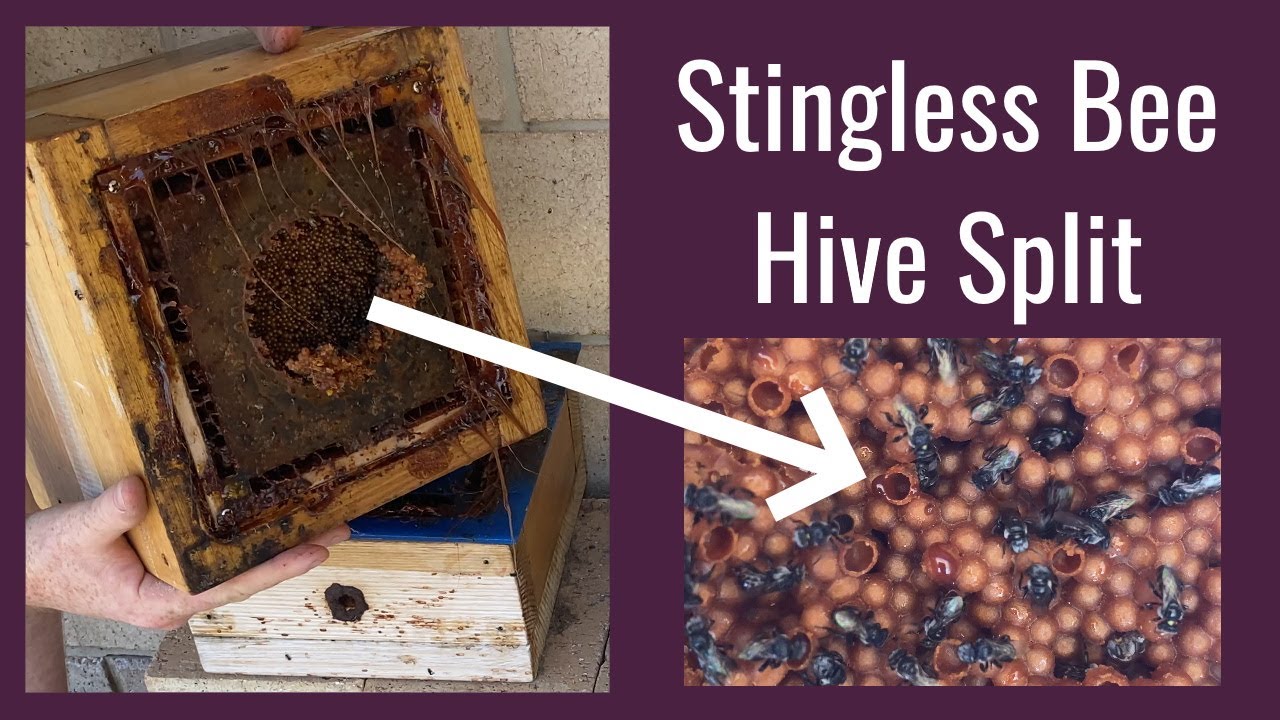The image features a detailed visual breakdown of a stingless bee hive split. The left side of the image displays a purple background with a white Caucasian man holding a wooden hive, which has been pulled apart to reveal an intricate honeycomb structure. Strings of goo and wax are visible within the square box that contains the hive. Below this, another squarish box with a blue interior houses another section of the hive. A white arrow points from the central portion of this left-hand image to the right side, which shows a close-up of the hive. In this close-up, we see a detailed view of the hive structure with predominantly closed cells, a few of which are open, allowing us to see bees crawling around. Above this close-up, the text "stingless bee hive split" is written in white. The right-hand image emphasizes the hive structure and the activity of the bees around it.